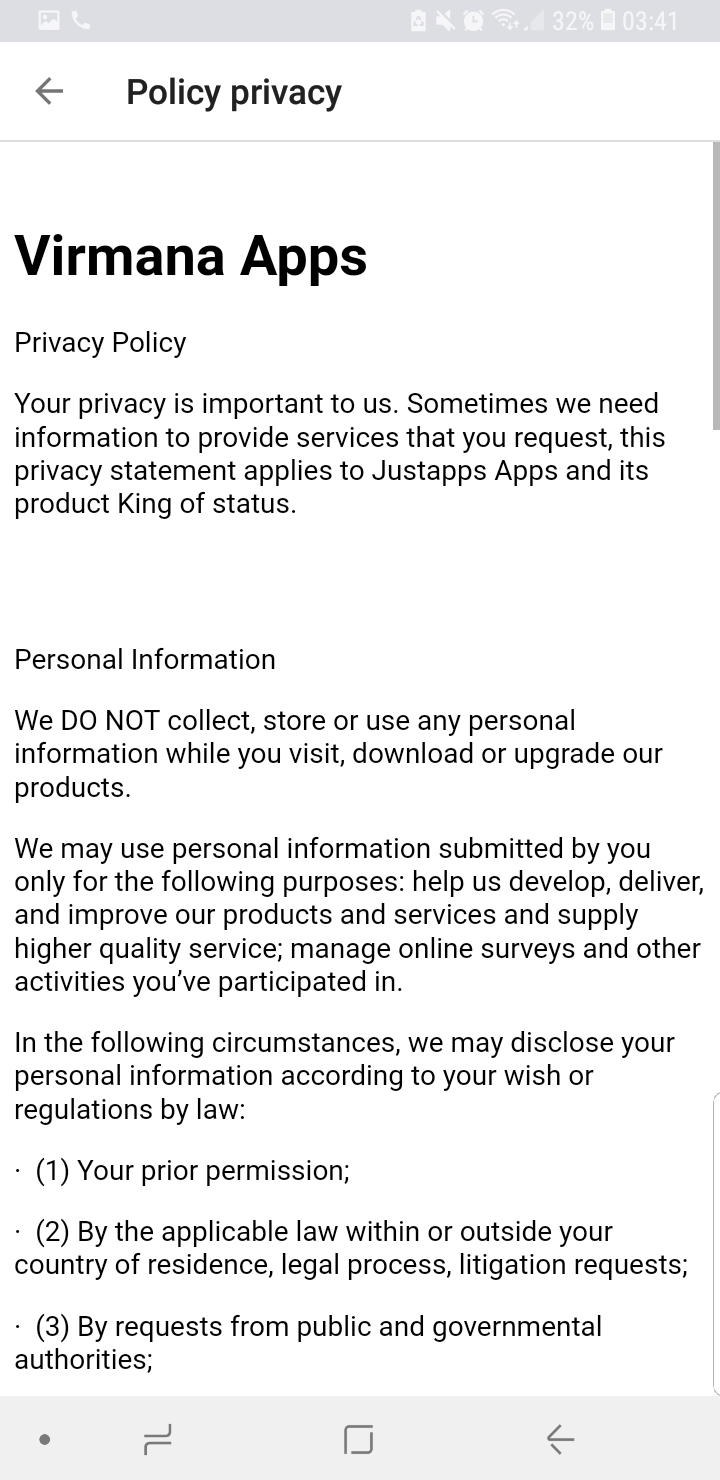**Detailed Descriptive Caption:**

The image displays a smartphone screen with a predominantly white background. At the top section of the screen, it is showing the device is currently charged to 32%. The time displayed on the phone is 03:41. Below the time, on the white background, there is a gray arrow pointing to the left, symbolizing a back navigation option. The word "Privacy" is inscribed in black beneath the arrow. 

Further down, there is a gray line followed by text that reads "Romana Apps Privacy Policy." A brief statement begins with "Privacy is important to us." This note indicates that at times information is required to provide requested services. The privacy statement applies specifically to the "Apps and its product King of Status."

The policy clearly states that no personal information is collected, stored, or used while visiting, downloading, or upgrading the products. However, it mentions that any personal information submitted by users is exclusively used for purposes like improving products and services, supplying higher quality service, managing online surveys, and other participatory activities.

Under specific circumstances, personal information may be disclosed according to user wishes or legal regulations. The points are itemized as follows:
1. With your prior permission.
2. By applicable law within or outside your country of residence, legal process, litigation request.
3. By request from public and governmental authorities.

At the bottom of the screen, in a gray area, there is another left-pointing arrow. Below this, there is a gray box, followed by two gray lines, and a gray circle, likely representing the navigation bar elements.

This elaborate depiction offers a comprehensive view of the privacy policy screen on a smartphone, with meticulous emphasis on textual content and graphical icons.